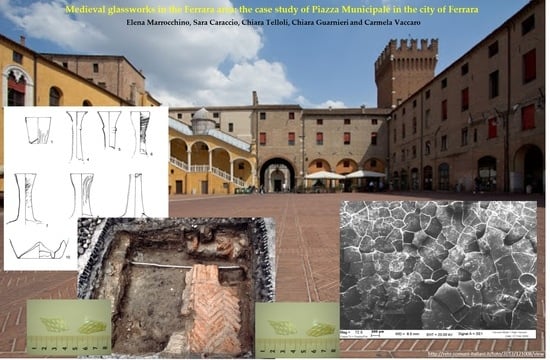This photo captures a detailed display of a historical analysis centered around a large, tan-colored medieval building situated in an open, rectangular city square that bears resemblance to castle walls. The photo, adorned with a title in bright yellow text reading "Medieval Glassworks in the Ferrara: A Case Study of Piazza Municipale in the City of Ferrara," attributes the work to Elena Maracino, Sara Caraccio, Chiara Tellelo, Chiara Guarmiera, and Carmela Vaccaro. Overlaying the main image are several additional photos and drawings that provide a comprehensive examination of the site and its glassworking history. 

On the left side, there is a precise, structural pencil drawing with a grid layout. Alongside it, two identical images depict green flecks of glass next to rulers measuring approximately three centimeters each, emphasizing the meticulous measurements involved in the study. In the center, we observe an excavated area, possibly a dig site for windows or glass remnants, showcasing half-exposed artifacts. To the right, a spectral analysis offers insights into the microscopic structural composition of the glass. These superimposed images collectively illustrate the detailed research and findings related to the medieval glassworks within the Piazza Municipale of Ferrara.